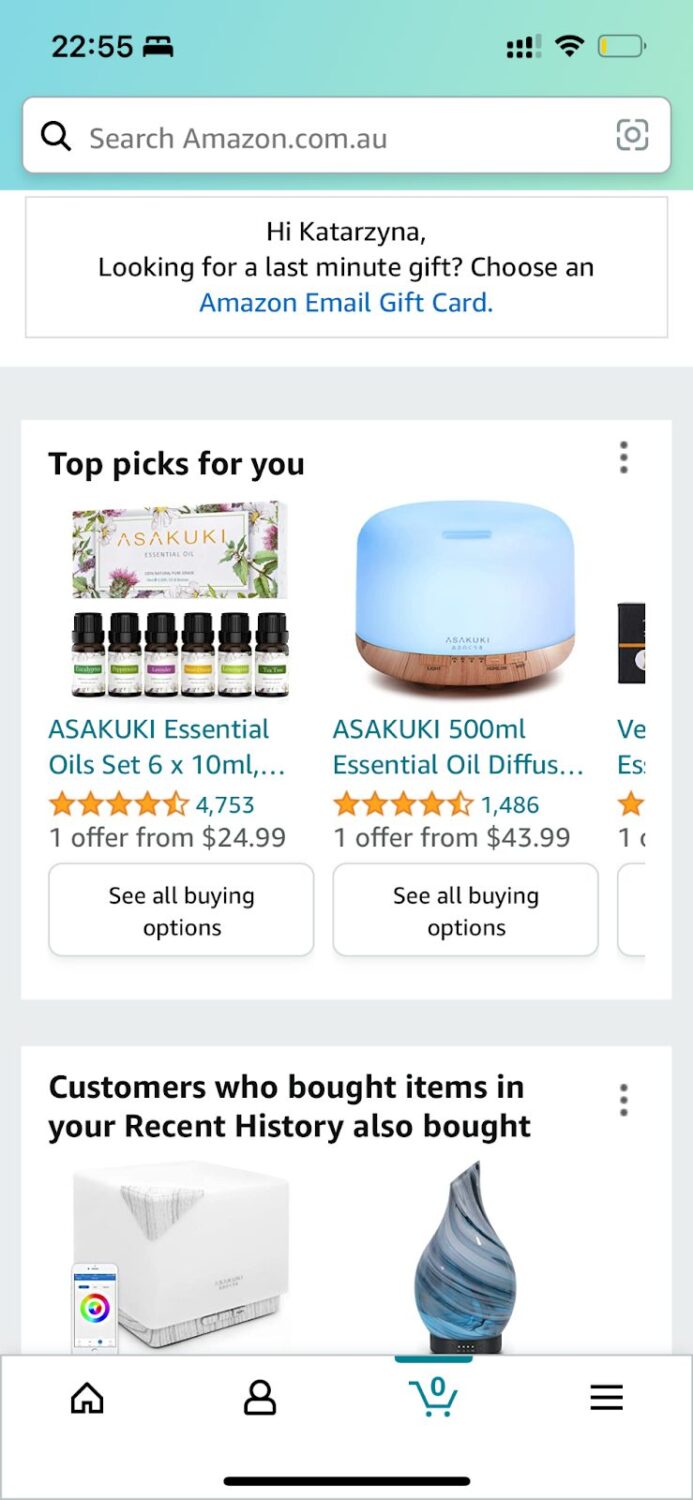A screenshot displays a webpage with a gray background taken at 10:20 pm. The URL in the search bar reads "amazon.com.au" accompanied by a magnifying glass icon on the left. A welcome message states, "Hi Katarzyna" followed by a suggestion: "Looking for a last-minute gift? Choose an Amazon email gift card." Below, there's a featured product section titled "Top Picks for You," showing an essential oil set and an essential oil diffuser.

1. **Essential Oil Set:** 
   - **Size**: 6 x 10 ml bottles
   - **Rating**: 4.5 stars (4753 reviews)
   - **Price**: One offer from $24.99
   - **Button**: "See All Buying Options"

2. **Essential Oil Diffuser:** 
   - **Size**: 500 ml
   - **Rating**: 4.5 stars (1486 reviews)
   - **Price**: One offer from $43.99
   - **Button**: "See All Buying Options"

Below these, another suggestion reads, "Customers who bought items in their recent history also bought," but no further products are displayed.